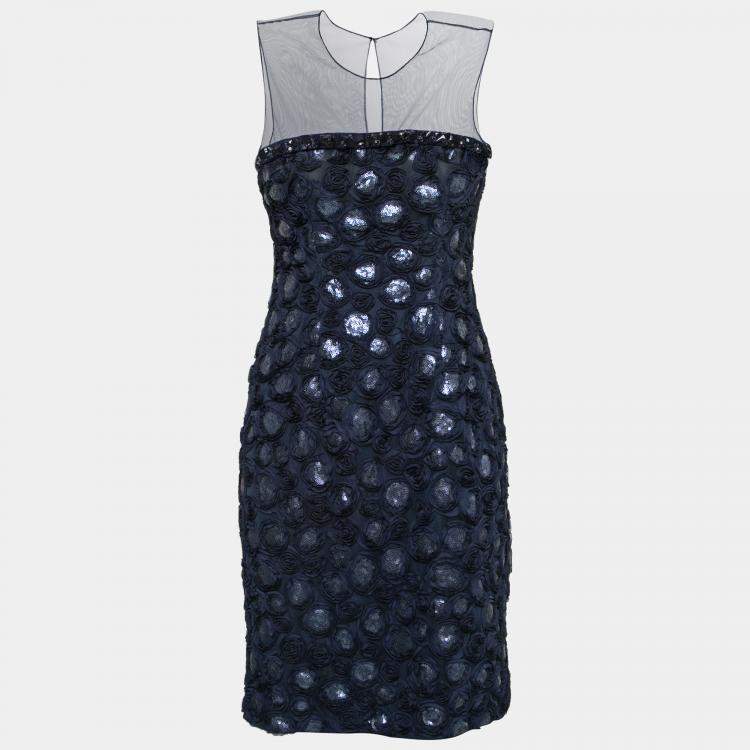The image showcases a sophisticated and elegant dress against a light gray, almost white, background. This sleeveless dress features a sheer, illusion top made of a gray or silver mesh that is transparent starting just above the bustline. The neckline is round and sits right at the neck. A shiny black band accentuates the upper section.

The main body of the dress transitions into a rich navy blue. Adorning the lower part of the dress are intricate, three-dimensional patterns resembling petals or scales, and some swirls that appear to be embroidered with metallic threads. Crystals are interspersed across the breast area and lower body, adding a shiny, reflective quality to the design. The dress is mid-length, reaching below the knees but not to the floor. The belly area cinches in, while the hip area flares out slightly, giving a flattering shape to the garment. The textured and reflective details of the dress convey a luxurious, almost ethereal aesthetic.